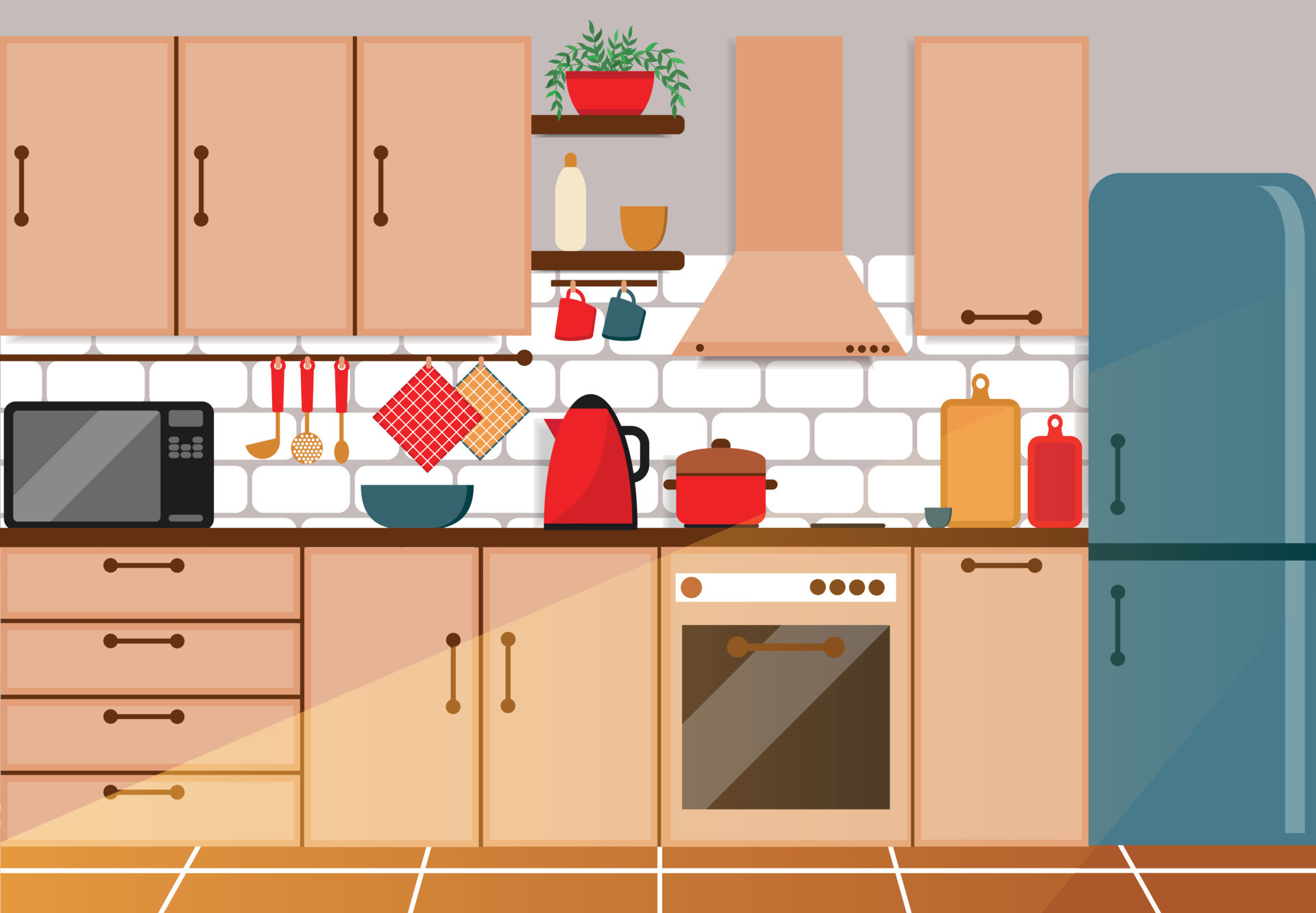This image is a detailed cartoon drawing of a kitchen. The kitchen features a brown tiled floor with white grout lines and is backed by white brick-style tile with gray grout. To the right, a blue, double-door refrigerator—freezer on the bottom and refrigerator on top—dominates the scene. Next to it, there’s a single cabinet with a handle and a pull-out drawer, leading to a peach-colored oven with a matching hood above it. On the left side of the oven, there are four under-counter drawers and a brown wooden countertop with a black microwave on top.

The kitchen is adorned with multiple items: a peach-colored pot with a lid on the stove, several utensils with red handles hanging underneath the cupboards, cutting boards, a blue bowl, coffee cups, and a possible water pitcher or large kettle. Above the counter, the cupboards—with brown drawer pulls—blend seamlessly with the peach color scheme. Additionally, hanging shelves hold various objects, including coffee cups, planters, and some bottles. The medium-gray walls above the backsplash frame the entire scene, adding depth and a touch of realism to this well-illustrated kitchen.